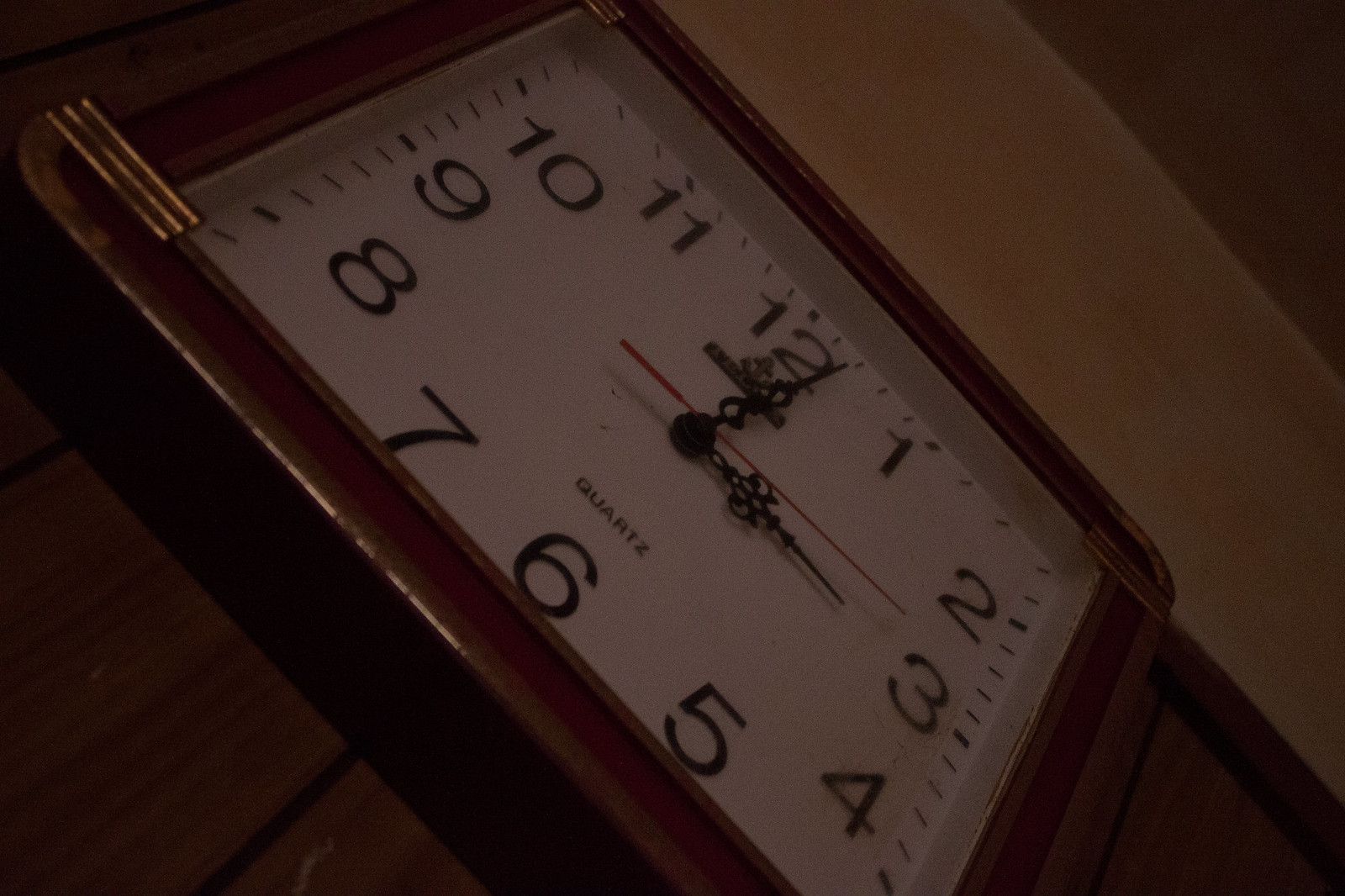This image features a distinctive square-shaped wall clock mounted on a brown wall, with the upper part of the wall being white. The clock has a white base and three central hands: a long, thin red second hand, and black hour and minute hands adorned with a delicate ribbon design. The clock face displays numbers from 1 to 12 in a traditional circular arrangement, with small black lines marking the minutes along the perimeter. The edges and corners of the clock frame are adorned with rectangular gold designs featuring intricate horizontal grooves, adding an elegant touch to its overall appearance.